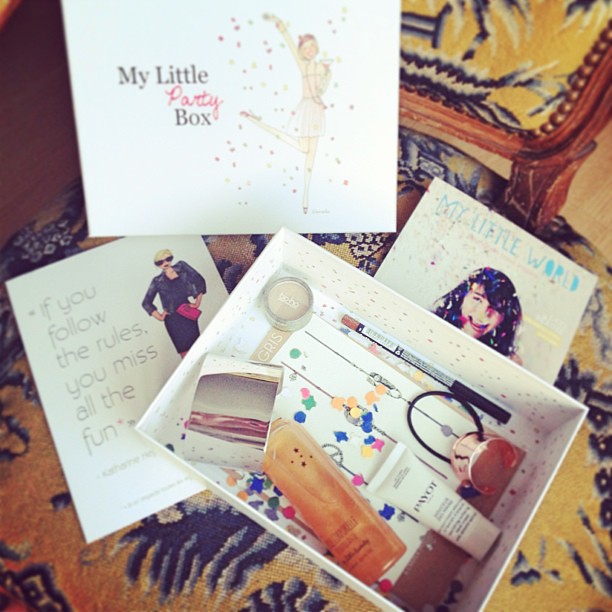The image displays four colorful advertisement cards resting on a floral-patterned cloth that evokes the vibrant, sometimes kitschy style of 60s and 70s furniture, characterized by its yellow and blue blossoms and leaves. At the top, a white square card titled "My Little Party Box" features an animated woman with one leg kicked up and an arm joyfully tossing confetti. Beneath her to the left, another card, "If You Follow The Rules, You Miss All The Fun," depicts a blonde woman in a black dress, holding a pink bag and wearing dark sunglasses. To the right side, there's a partially visible card titled "My Little World," showcasing another woman's face adorned with confetti. At the bottom center of the image, a box containing several makeup items, including a brush and various bottles, lies open. The photograph appears to be captured from a top-down perspective, revealing parts of what might be a purse or suitcase with brown beadwork in the upper right corner.